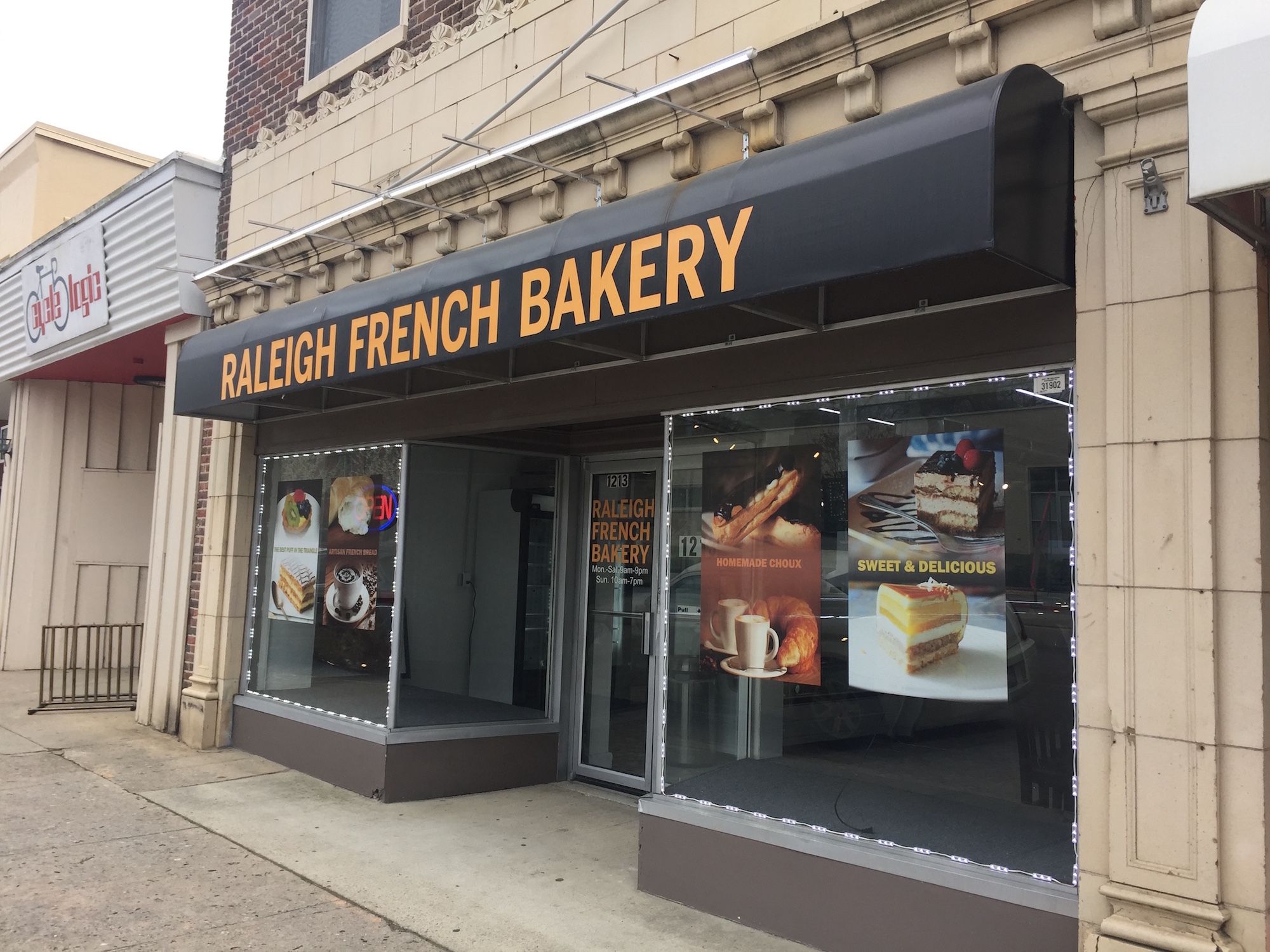The image is a color landscape photograph of a city street featuring a storefront at an angle. The main focus is the Raleigh French Bakery, prominently marked with bright yellow block letters on a black canopy overhead. The bakery's door, centrally positioned, also bears the bakery's name and the street number 1283. Flanking the door, there are two window displays showcasing an array of baked goods, including a croissant, an éclair, a piece of tiramisu cake with the label "sweet and delicious," and cups of drinks. The bottom of the store windows is dark brown, while the building itself is topped with brown brick and beige concrete blocks.

Adjacent to Raleigh French Bakery is another business identified by a white sign with red letters reading "Psychologic," indicating a bicycle shop. This shop features a wall rack for bikes and a bike logo prominently displayed. The angle of the photograph captures a portion of the gray sidewalk in front of both stores. The overall scene reflects a lively and inviting city street, framed in the style of photographic representational realism.